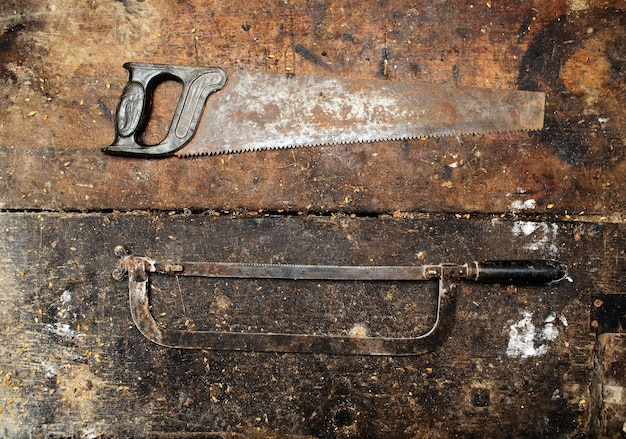The image features two distinct, old, and worn tools lying on a stained and weathered wooden bench with splatters of white paint. The upper half of the picture depicts a traditional hand saw, characterized by its wide, tapering silver blade, which narrows towards the brown handle. The jagged teeth of the saw are prominently positioned along the bottom edge of the blade. The handle, designed for grip, appears to be slightly rusted and timeworn. The lower half showcases a hacksaw with a straight blade running from its black handle, arcing towards the end and supported by a metal frame that mirrors the blade's shape. Both tools display significant signs of rust and age, giving the impression they haven't been used in quite some time. The worn surface of the bench further enhances the rustic and nostalgic feel of the image.